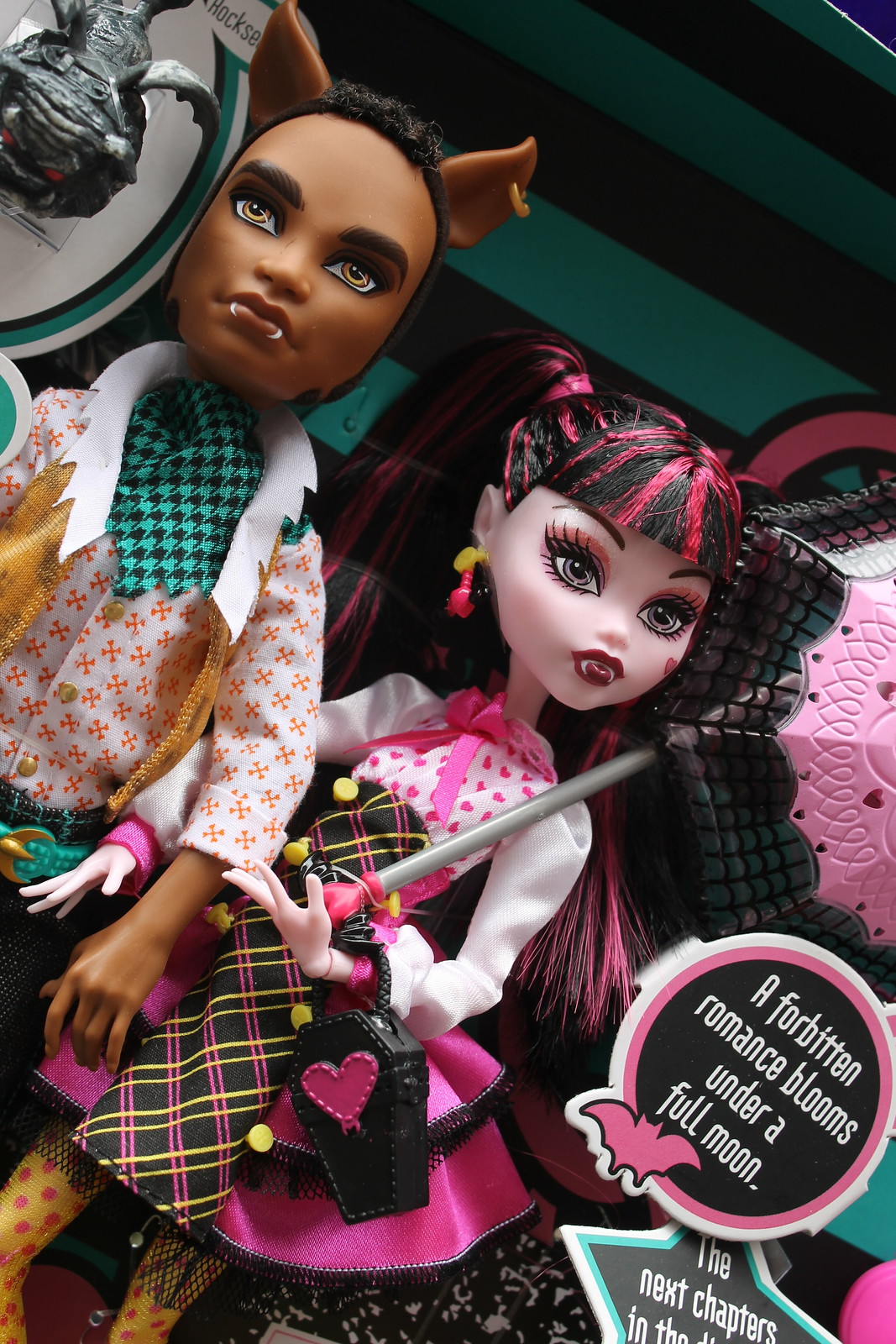The image shows two non-traditional dolls posed at a slant to the right. The male doll, on the left, is dark-skinned with large, animal-like ears and small fangs. He has white eyes and wears a turquoise and black checkered shirt with a rough white collar and an overlay jacket with yellow accents. He also has a turquoise belt at his waist. The female doll, on the right, is light-skinned with pink and black hair styled with bangs. She has large eyes and small fangs at the corners of her lips. Her attire consists of a white blouse with tiny hearts, a pink collar, a pink tie, and a pink skirt. She wears yellow stockings with polka dots and holds a black coffin-shaped handbag with a pink heart. Additionally, she carries a parasol in her left hand, featuring a spiderweb design. Completing the scene is a sign that reads, "A forbidden romance blooms under a full moon," accompanied by a black circle with a pink bat and a star graphic, followed by the partial phrase, "The next chapter."